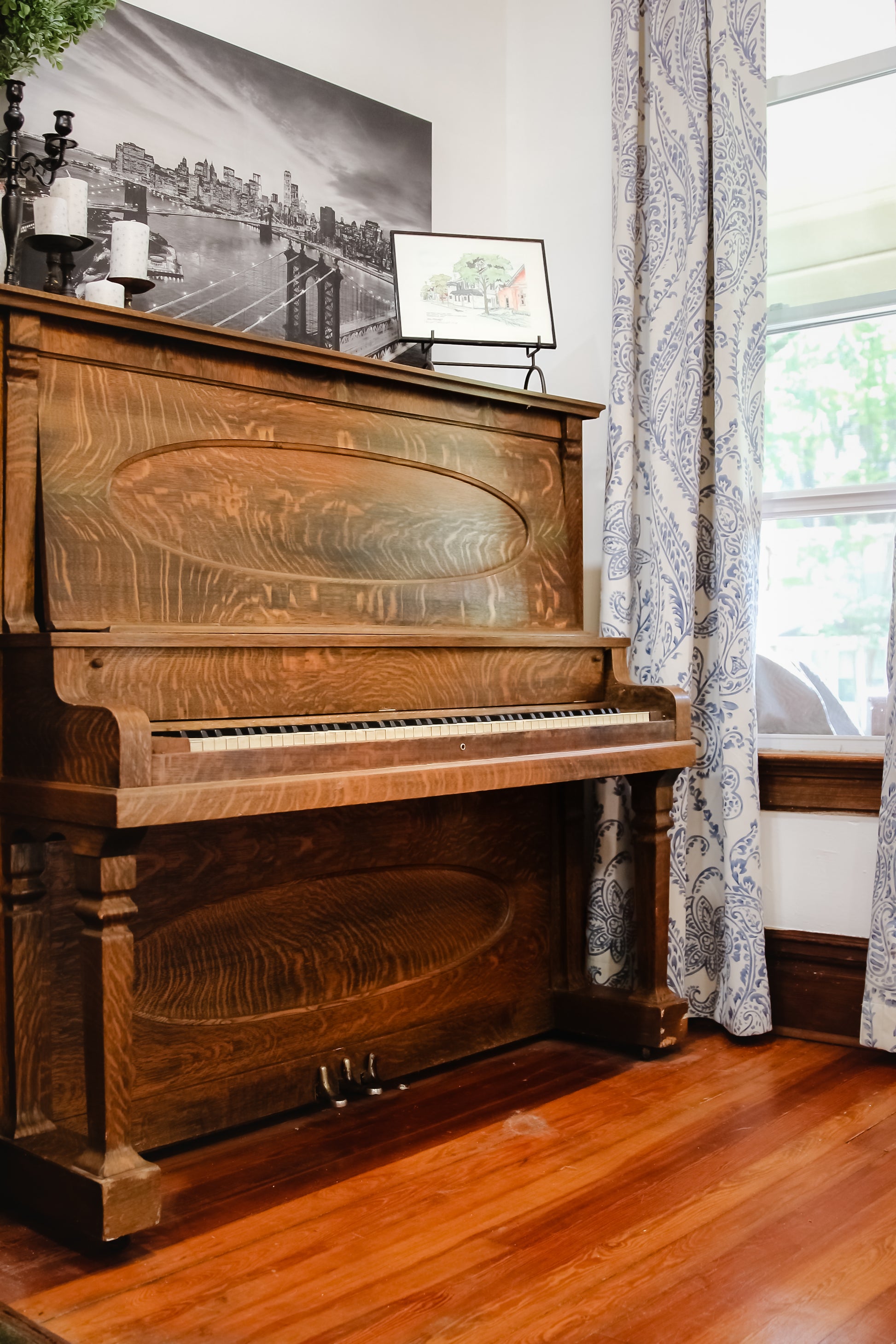This image depicts a vintage wooden piano positioned against a white wall with a window. The window is adorned with curtains that feature a delicate white and light blue filigree design. The piano, which has white and black keys along with three metal pedals at its base, stands on a rich brown hardwood floor. On top of the piano, various items are displayed, including a small painting in a black frame with a cartoon-like graphic of trees and a building, candles, and a candle holder. Also atop the piano is a black and white photograph showcasing a city skyline with a suspension bridge, evocative of the New York City skyline with the Manhattan and Brooklyn Bridges. The right side of the scene reveals a view through the window of sunlit green trees, framed by the wooden borders of the window. Notably, there is no seating available near the piano.